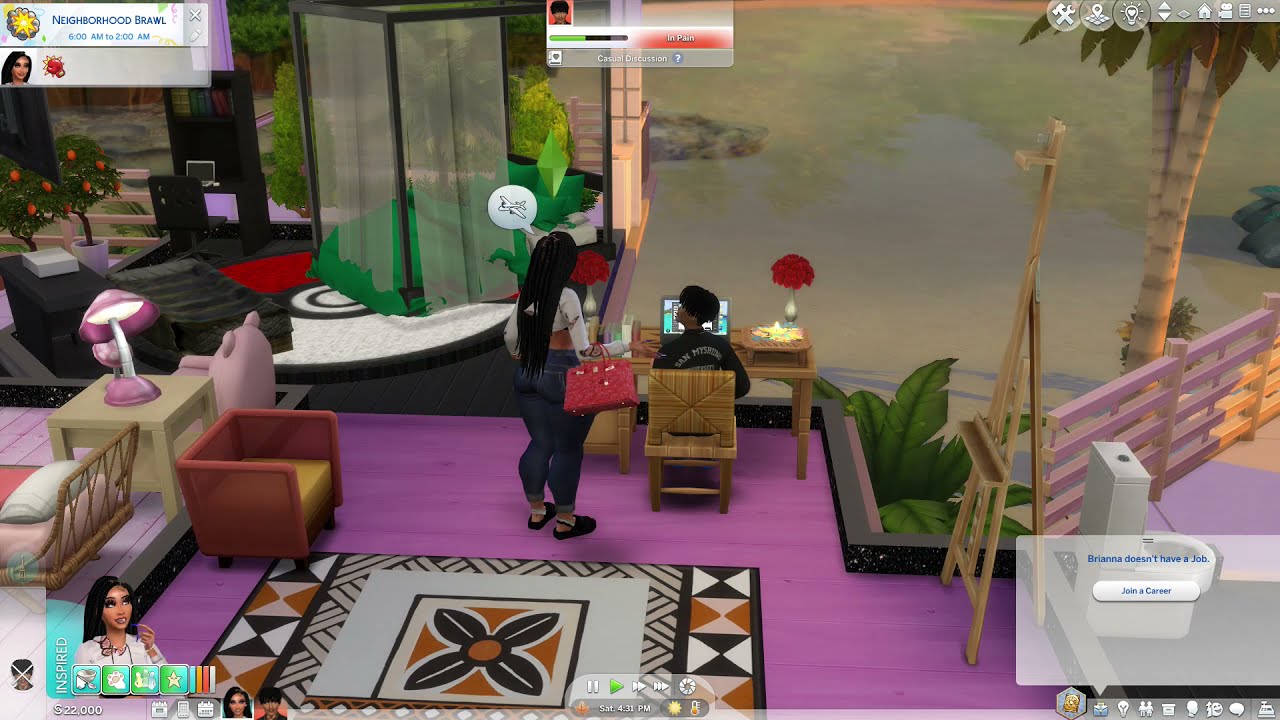The image is a screenshot from a simulation video game, possibly similar to The Sims. The upper left corner features a text box with the label “Neighborhood Brawl,” and lists the event time as “6 a.m. to 2 a.m.” Below this text box, there is a female avatar adjacent to a red icon. Dominating the center of the image is a woman with long dark hair, clad in a white shirt, blue jeans, and black shoes, holding a red handbag. She stands next to a desk where a man with black hair, styled in an Afro, is seated, facing away from the viewer. The man's desk setup includes a laptop and a white vase containing red roses. The desk and the characters are positioned on a pink floor, partially covered by a large rug with brown and black geometric patterns interspersed with orange and white floral designs.

To the left of the woman, there is a reddish chair with a yellow cushion, accompanied by a small table that holds a lamp. In the broader room context, an array of additional furniture and items populate the space, such as another chair under draperies and what appears to be an easel for painting to the right. There is also a pink staircase and a pink gate visible. The background features an orange tree or fruit-bearing bush, and what resembles a shower stall can also be discerned. On the right side of the screen, a text box pops up indicating, “Brianna doesn’t have a job” with an option to “join a career,” underscoring the game’s simulation nature.